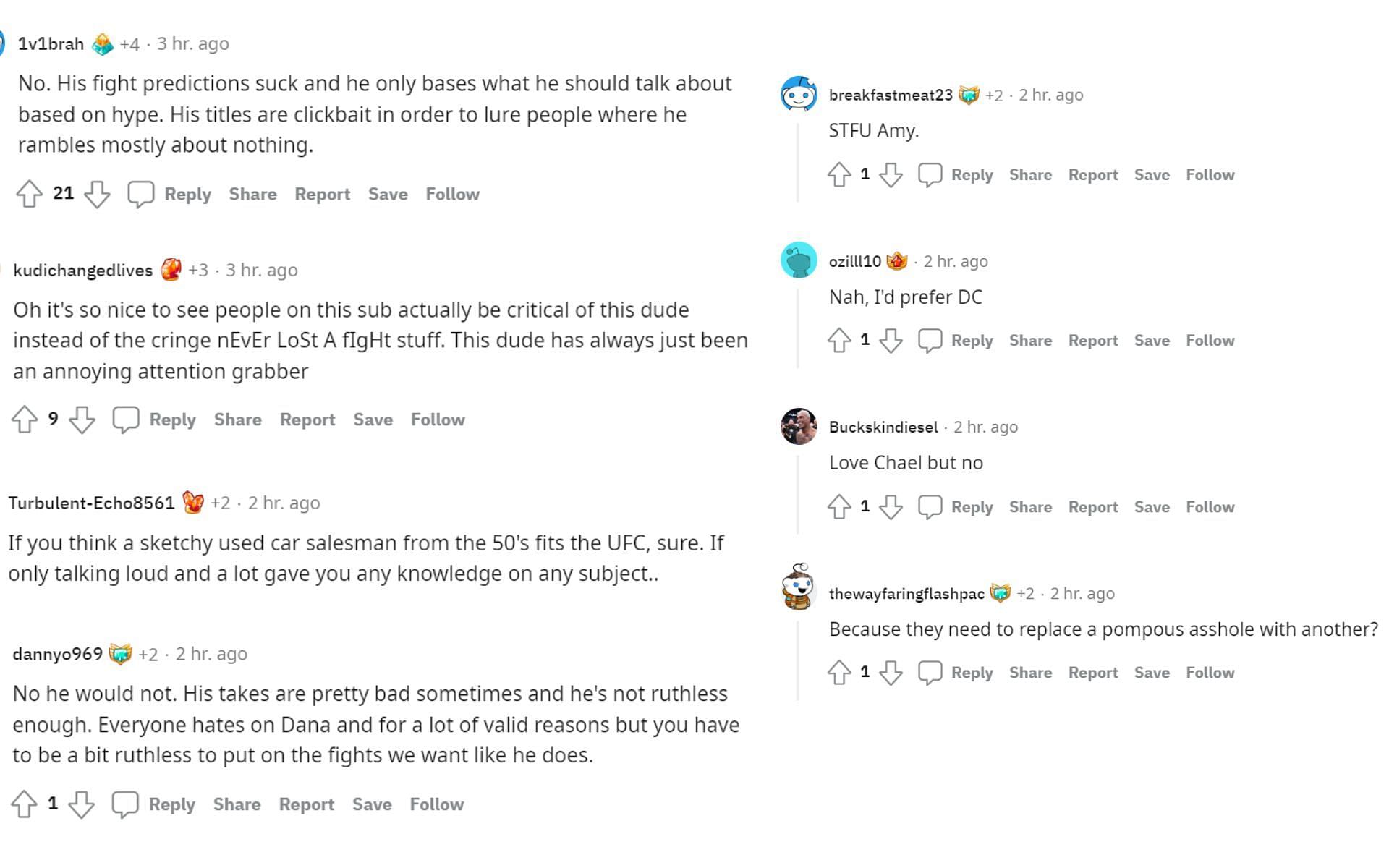This Reddit post captures a lively discussion regarding a controversial figure in the UFC community. The post has amassed nine comments, each contributing to a heated debate. The first comment criticizes the figure for making poor predictions based purely on hype, using clickbait titles, and often rambling about women. This comment has received 21 upvotes. Another user appreciates the critical perspectives on the subreddit, noting that it’s a refreshing change from the usual uncritical or 'cringe' content. This user views the figure as annoying and attention-seeking, likening their demeanor to a sketchy 1950s used car salesman. The thread also includes terse interactions, such as one commenter telling another to "shut the fuck up," and a brief discussion on preferences for a different commentator, "DC," who is compared favorably to the contentious figure. Overall, the comments reflect a diverse range of opinions, from critical to supportive, highlighting the polarizing nature of the individual in question.